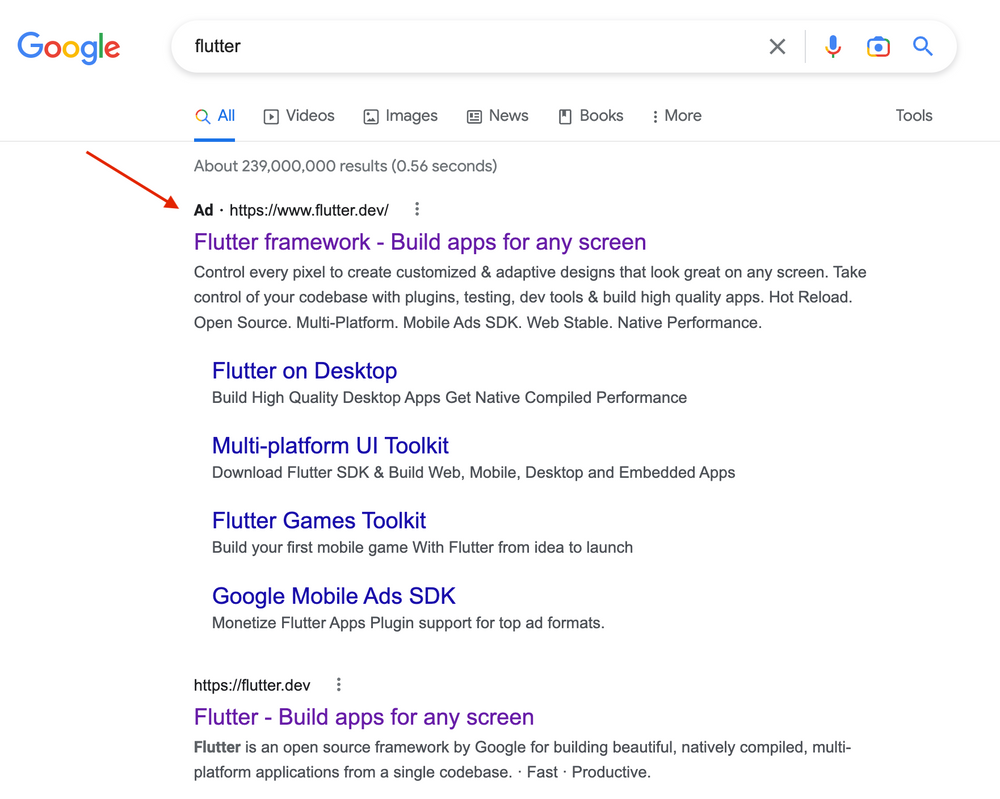**Detailed Descriptive Caption:**

The screenshot captures a Google search results page. In the upper left corner, the colorful Google logo is prominently displayed, with the capital 'G' in blue, followed by a small 'o' in red, another small 'o' in yellow, a small 'g' in blue, an 'l' in green, and a small 'e' in red. To the right of the logo is the search box containing the word "flutter". Adjacent to the search box's right edge is an 'X' icon, followed by a microphone icon, a camera icon, and a magnifying glass icon.

Directly below the search box, a navigation row features a multi-colored magnifying glass icon beside the word "All", indicating the active tab, underlined by a blue line. Additional options in this row include "Videos", "Images", "News", "Books", and a menu accessible via three vertical dots labeled "More". At the right end of this row is the word "Tools".

Below these navigation options, a status phrase indicates "About 239,000,000 results (0.56 seconds)" in numerals. This is followed by a listing that begins with the word "Ad" in purple text, next to the URL "https://www.flutter.dev", and three vertical dots. A superimposed red or yellow arrow points diagonally to the word "Ad" from the left.

The primary search result headline is "Flutter Framework - Build Apps for Any Screen" in purple, suggesting a previously clicked link. The snippet beneath it reads: "Control every pixel to create customized and adaptive designs that look great on any screen. Take control of your code base with plugins, testing, dev tools, and build high-quality apps. Hot reload, open source, multi-platform, mobile ads, SDK, web stable, native performance."

Further down, the page presents hierarchical bullet points: 
- "Flutter on Desktop"
  - "Build high-quality desktop apps, get native compiled performance."
- "Multi-Platform UI Toolkit"
  - "Download Flutter SDK and build web, mobile, desktop, and embedded apps."
- "Flutter Games Toolkit"
  - "Build your first mobile game with Flutter from idea to launch."
- "Google Mobile Ads SDK"
  - "Monetize Flutter apps with plug-in support for top ad formats."

The subsequent result repeats the pattern of the URL "https://www.flutter.dev" followed by three vertical dots. The headline "Flutter - Build Apps for Any Screen" links to a new description stating: "Flutter is an open source framework by Google for building beautiful, natively compiled, multi-platform applications from a single code base. Fast. Productive."